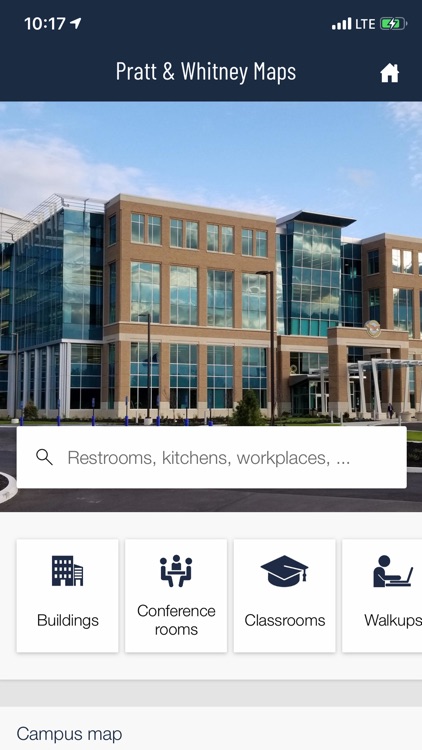The image displays a cell phone screen showing various elements related to Pratt & Whitney Maps. At the top, the phone's status bar indicates the time as 10:17, an LTE connection with full reception bars, and a green battery icon denoting the device is charging. Below the status bar, the screen header reads "Pratt & Whitney Maps" in white font against a black background, accompanied by a small house icon symbolizing the homepage.

Beneath the header is an image of a three-story office building with numerous windows, set against a backdrop of a clear blue sky. Below this photograph, there is a white search bar with a magnifying glass icon and placeholder text that reads "rooms, kitchens, and workplaces..."

Further down, on a white background, are four rectangular buttons with varying shades of white. Each button has an icon and a label: 
1. "Buildings" with a building icon. 
2. "Conference Rooms" with an icon of three people sitting at a table.
3. "Classrooms" with a graduation cap icon.
4. "Walk-ups" with an icon of a person working at a laptop, though the text is partially cut off.

At the bottom of the screen, a darker gray bar contains a label that reads "Campus Map." The dominant colors on the screen are black, white, and gray, contributing to a clean and professional look for the Pratt & Whitney Maps interface.